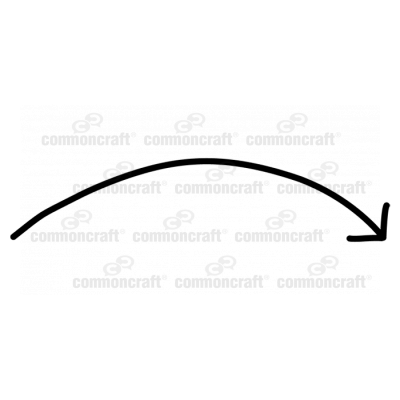This image features a digitally-created graphic with a prominent black arrow and a subtle watermark. The arrow, which starts on the left and arches over the center, ends on the right with its tip pointing downwards. The background is primarily white, with shades of light gray, darker gray, and black adding contrast. The only text in the image is the watermark "Common Craft," positioned discreetly behind the arrow in a very light gray or silver print. The arrow is centrally positioned in relation to the watermark. This image could be used as clipart or a graphic on a website, requiring appropriate usage permissions.